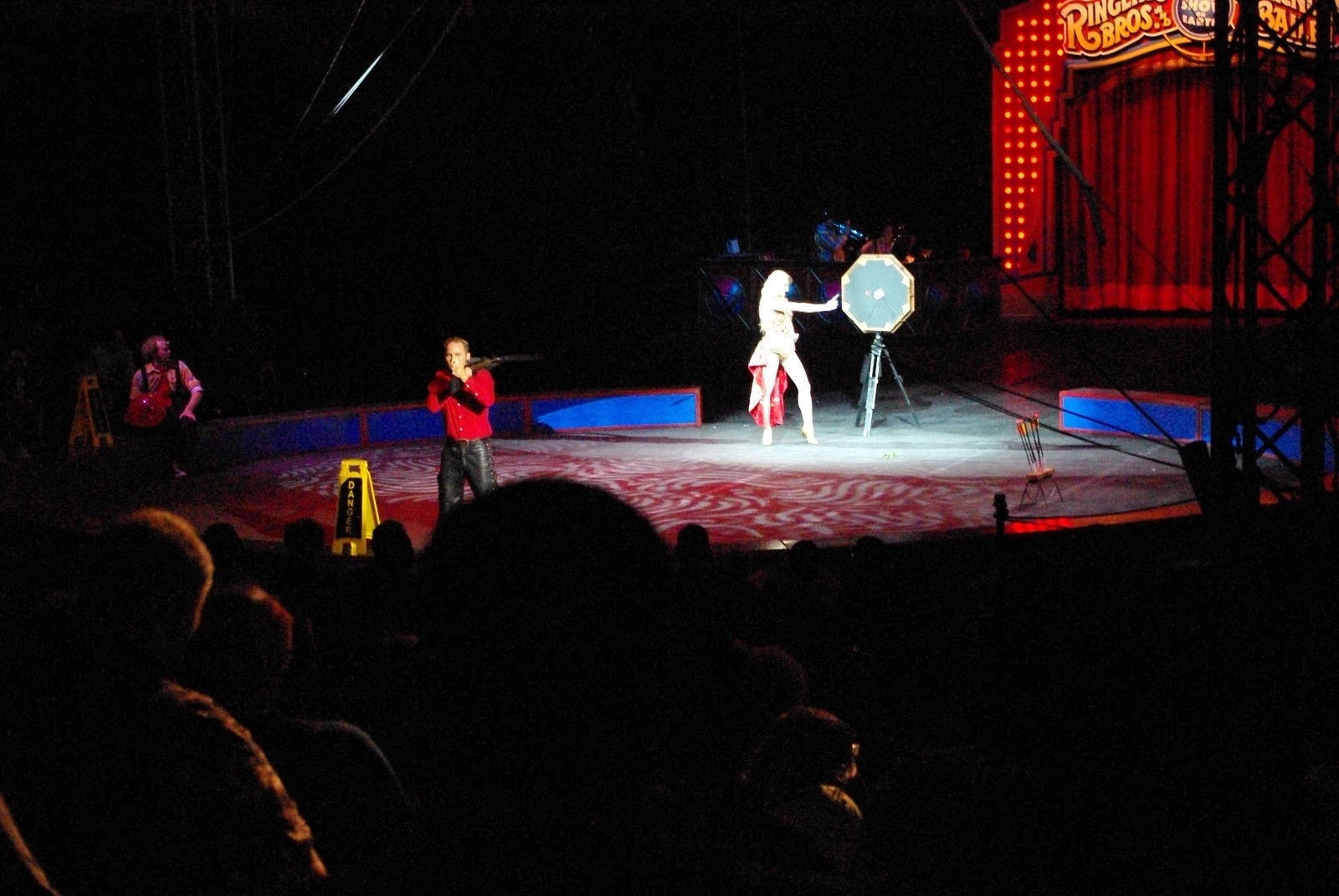The full-color photograph captures an indoor circus performance, identifiable by the "Ringling Brothers" sign prominently displayed in the upper right-hand corner. The perspective seems to be from the audience, with silhouettes of crowd members visible in the foreground, illuminated only minimally by backlighting. On stage, under the spotlight, is a dramatic scene: a man in black pants and a long-sleeved red shirt, potentially holding a crossbow or a microphone, is positioned center-stage. To his right, about twelve feet away, stands another man in a lighter shirt, looking ahead. 

Dominating the background, a woman in a sexy, short white outfit with her full legs showing stands in front of a pedestal that holds a round, blue object adorned with yellow or white dots around its circumference. This object, potential a target board, suggests she is part of an act involving either thrown or shot objects, alluding to the possibility of her being part of a daring crossbow performance. The stage itself is decorated with a reddish carpet, and a yellow caution-like stand adds a splash of brightness to the vivid scene.